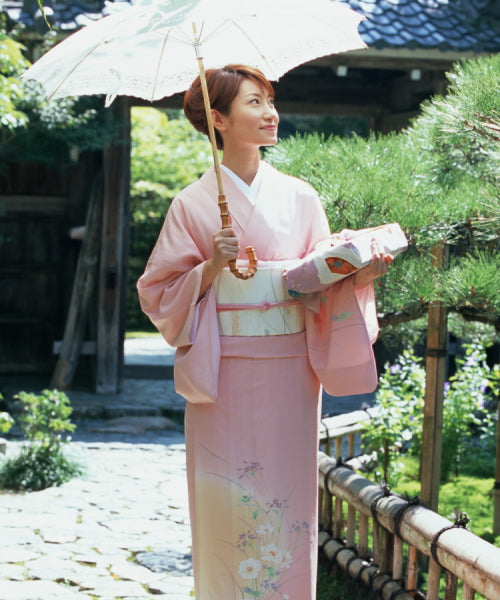The image showcases a beautiful young Japanese woman with auburn hair elegantly tucked behind her head, with a few bangs falling gently on her forehead. She is adorned in a pistil pink kimono that features a white band around her waist, large sleeves, and intricate floral designs at the hem. The woman is holding a delicately wrapped present in one hand, matching her kimono's hue, as well as a dainty white umbrella with lacy edges that curves at the bottom.

She's standing in a picturesque garden bathed in sunlight, highlighting the lush green plants and casting a warm glow on her serene surroundings. A short wooden fence borders some trees, enhancing the garden's quaint charm. The woman is front-facing but looking up and to the right with a gentle, closed-mouth smile, giving her an air of contentment as she gazes at something in the distance. The overall scene evokes a sense of tranquility and cultural elegance, capturing a moment of grace and beauty in a traditional Japanese setting.